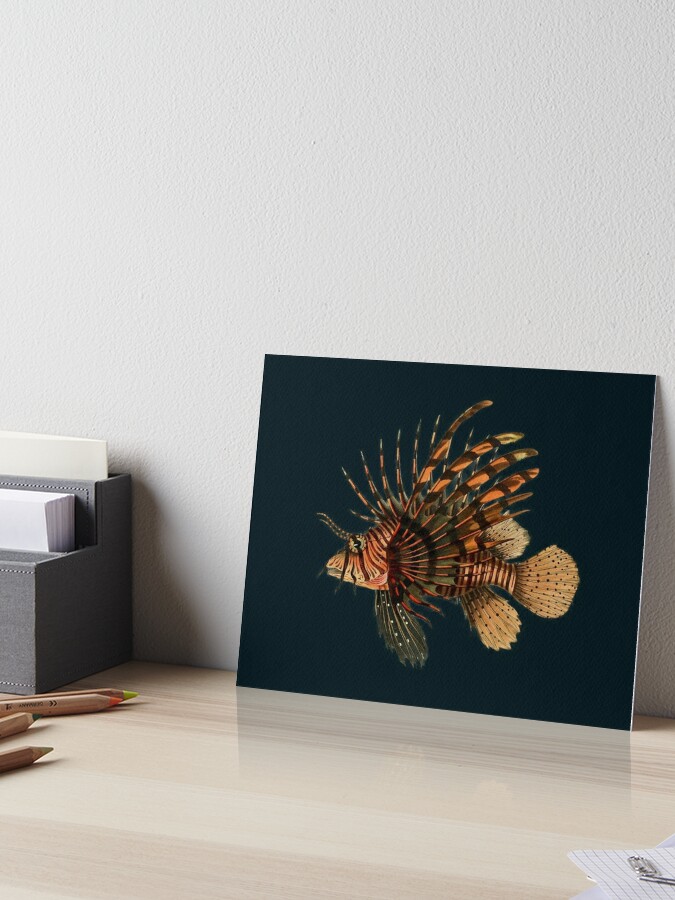The image showcases a stunning art print of an orange and black lionfish, set against a dark background, prominently displayed on a wooden or glossy pine desk. The detailed fish features seven distinct spikes protruding from the front of its body, with longer, feather-like tendrils extending from its back. The lionfish's intricate coloration includes vibrant oranges and browns, with beautiful orangey spikes, darker fin underneath its mouth, and light orange tail fins. Accompanying this piece are various drawing tools—pencils scattered to the left side of the desk, and a few papers and paper clips within an organizer. The art print is a vivid portrayal, blending striking patterns of stripes around the fish's face and polka dots trailing along its fins, creating an impression that evokes the mysterious allure of deep ocean life.